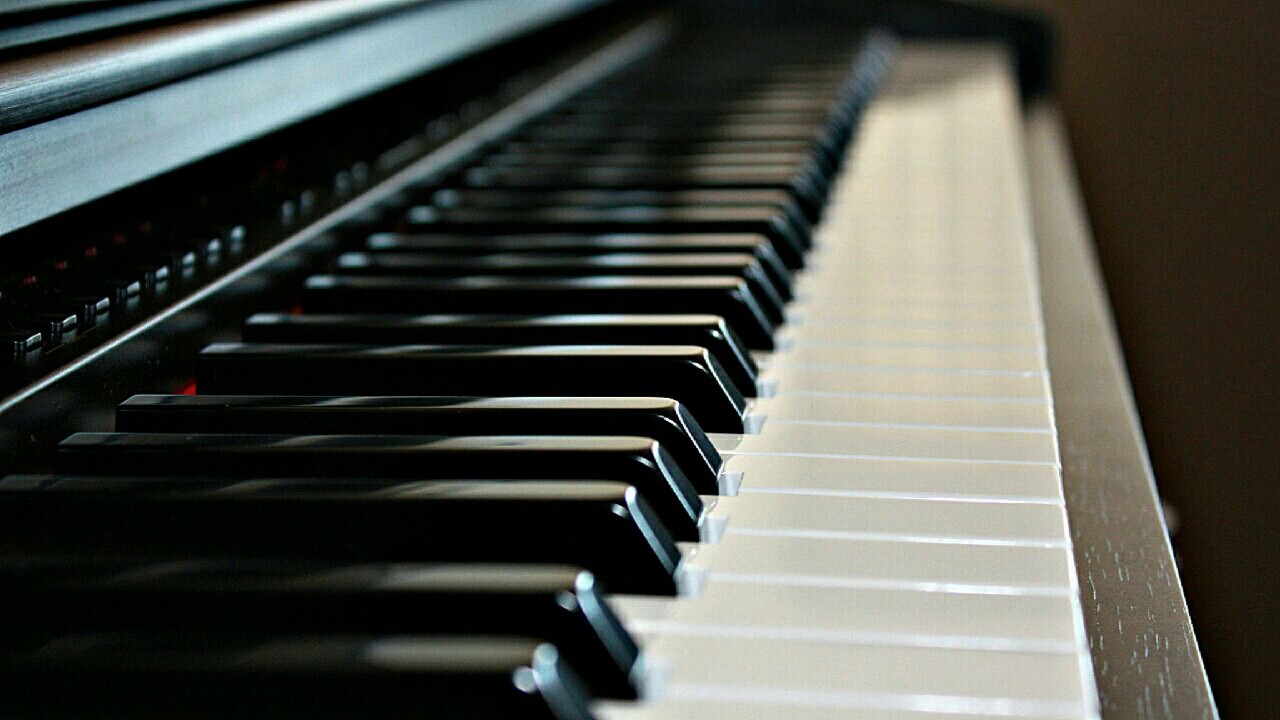This image is a close-up photograph of a digital piano taken from a low angle, where the focus is primarily on the white and black keys. The keys, arranged in neat rows, span the entire front bottom portion of the image and appear to stretch out into the distance, gradually becoming out of focus towards the top. Buttons and controls are visible along the left middle and extending into the center of the frame, indicating the digital nature of the piano. A red light, likely the power indicator, is illuminated in the middle section above the keys. The top portion of the photograph includes a blurred view of the piano's facade, which reveals a wood grain texture along the right-hand side, adding a touch of classic elegance to the modern instrument. The black keys are notably shiny, reflecting light and adding contrast to the more matte appearance of the white keys.